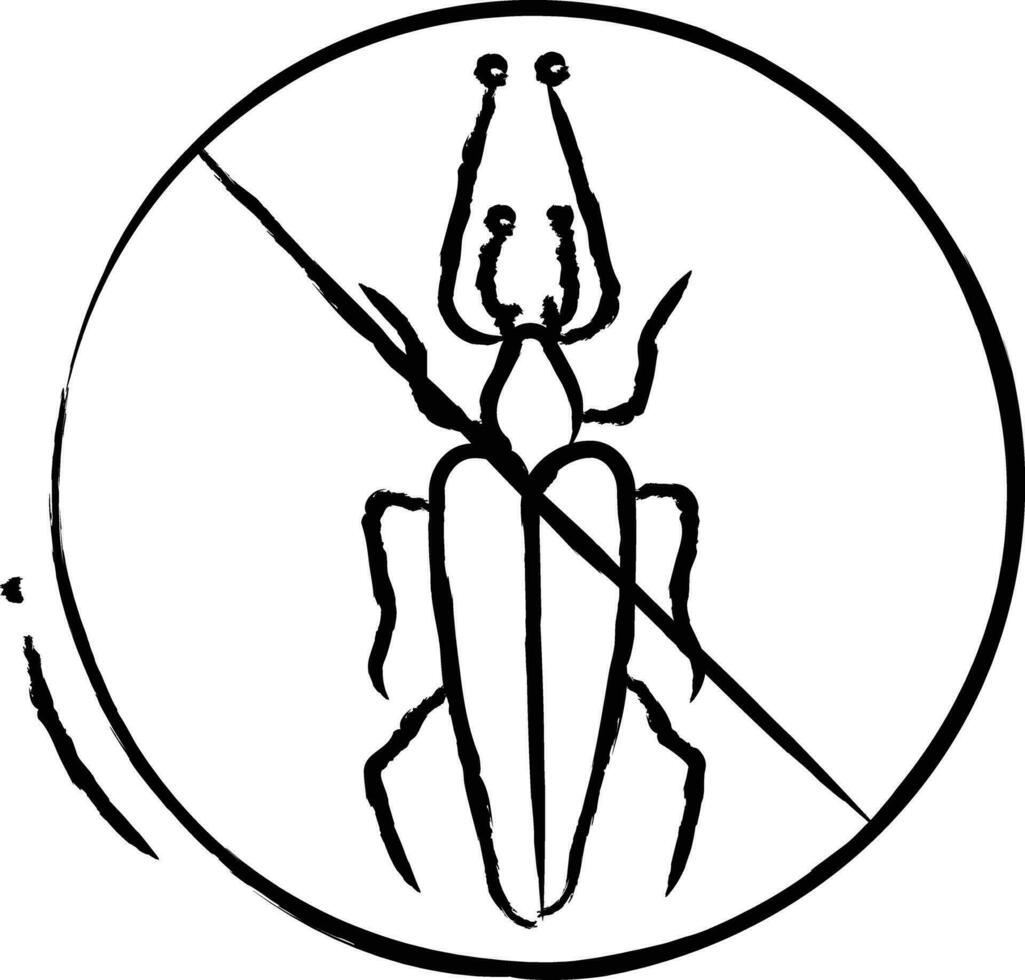This image features a detailed, hand-drawn, black-and-white logo depicting an insect, appearing to be either a beetle or a cockroach. The insect is oriented facing upward, with a large, segmented abdomen composed of two long shell halves, and is depicted as a precise line drawing. It has six legs, with two sets of antennae: a small inner set and a larger outer set. The insect is enclosed within a black circle with a prominent diagonal slash running from the upper left to the lower right, symbolizing a prohibition, akin to a "no bugs" sign. The background is white, further highlighting the stark black ink of the drawing. Additionally, there is a black arc outside the circle in the bottom left corner, mirroring the circle's shape. The simplicity and monochromatic nature of the drawing, possibly created with a marker, suggests it could serve well as a logo or even a button.